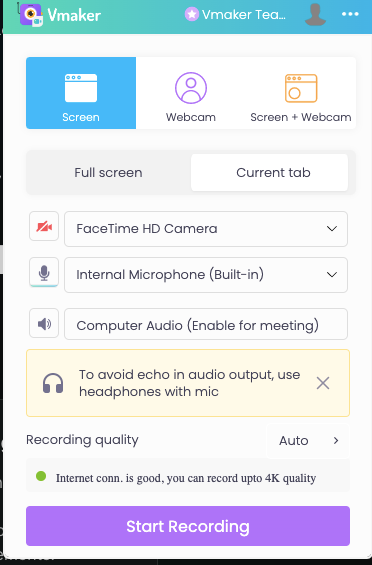This image, captured from a cell phone, displays the interface of a V-Maker application, likely a video creation tool. The screen prominently features a partially visible title, "V-Maker T-E-A...," which might suggest "teacher" or another similar term. Dominating the interface, a gray silhouette of a human figure is situated near the top right, accompanied by three white dots, possibly indicating a menu or options.

At the top of the screen, there are three selectable options: "Screen," "Webcam," and "Screen & Webcam." The "Screen" option is currently highlighted in a blue rectangle, indicating it is the active selection. To the right of this, the "Webcam" option is marked with a purple circle bearing a person icon, whereas the "Screen & Webcam" option is distinguished by an orange rectangle featuring a composite icon of a screen and circles.

Moving down the interface, there are options labeled "Full Screen" and "Current Tab," with "Current Tab" selected. Additional settings display "FaceTime HD Camera" and "Internal Microphone (Built-in)," accompanied by icons of a camera with a line through it and a microphone, respectively. This section ensures users are aware of their audio and video input options.

Further down, a speaker area labeled "Computer Audio Enabled for Meeting" suggests audio settings, followed by a recommendation to use headphones with a microphone to avoid echo in audio output. At the very bottom, a prominent purple box labeled "Start Recording" beckons the user to initiate their video capture.